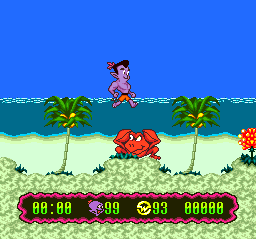A vibrant gameplay scene set on a picturesque sandy beach. In the foreground, tan-colored sand stretches across the bottom of the image, adorned with colorful graphics in shades of pink, green, and brown. A prominent timeout timer displays "0:00." On the left side of the screen, a purple-faced creature with a green "99" above its head is seen, accompanied by a gold icon with the number "93." Below these, multiple zeros line up along the bottom of the screen.

Flanking the scene are two palm trees with leaves in various shades of green, yellow, and tan, framing a red crab with an angry, frowning expression and upraised claws. In the background, a genie-like character treads on water, showcasing distinctive features such as purple skin, black hair, pointy ears, and red swim trunks. The sky above is a clear blue, and the ocean is a mesmerizing teal adorned with white-tipped waves, completing this vivid seaside tableau.